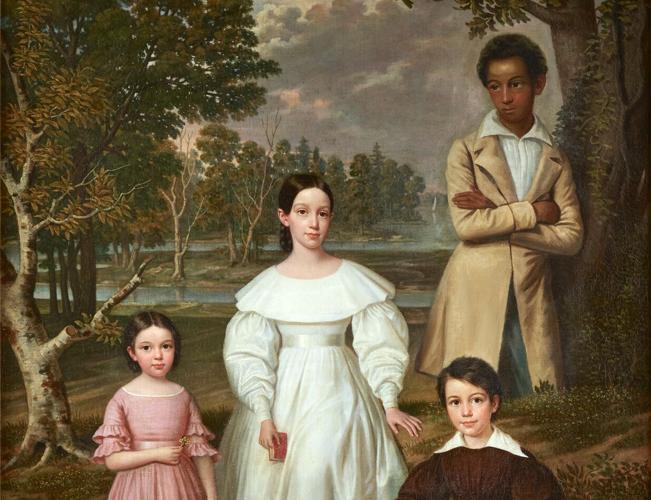This detailed painting captures a serene outdoor scene, seemingly from the early 1900s, with four focal characters amidst a lush and colorful landscape. Central to the composition are three children and a young man. On the far right, a tree with brown, orange, and green leaves stands prominently, accompanied by another tree in the background. In the foreground, a little girl with short brown hair and light pink skin dons a pink dress with ruffled sleeves. Beside her, a taller young woman, or possibly an older girl, wears a striking white dress with ruffled sleeves, a white ribbon around her waist, and a white collar, her brown hair styled in a braid or bun. To her other side stands a young boy in a brown shirt with a white collar, his light skin and brown hair accentuated by his bright smile. Behind them, leaning against a thick tree surrounded by abundant vegetation, is a young black boy with a short afro and rosy pink cheeks. He wears a white shirt with a white collar under a tan blazer, standing with his arms crossed and looking pensively into the distance. The background features more trees and a tranquil pond under a slightly cloudy sky. The painter’s skill is evident in the detailed, professional quality of this captivating scene.